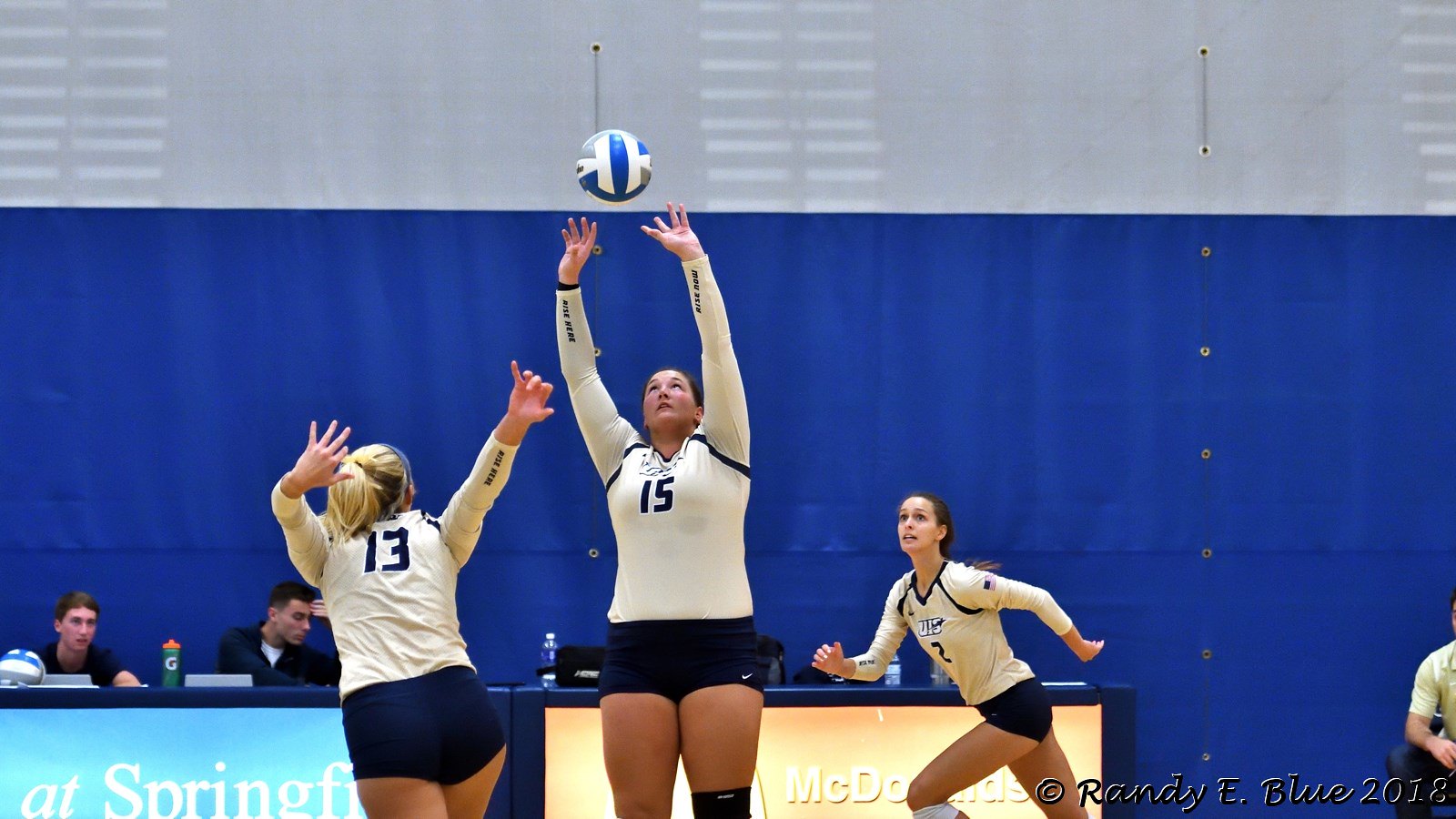In this detailed image, a dynamic scene from a competitive indoor volleyball match is captured. The photograph prominently features three young female players with fair skin and blonde hair, all clad in white long-sleeve jerseys and blue shorts. Centered is player number 15, reaching upward with the volleyball nearly in her hands, poised to set it. To her left, player number 13 is seen from the back, her arms trailing as she races toward the ball. Meanwhile, to the right, a girl with darker hair and jersey number 2 is sprinting forward.

The backdrop is dominated by a blue and gray divider net adorned with grommets, occupying a substantial portion of the upper three-fourths of the image. Below this divider, the scorer's table, situated off-center to the left, features two male individuals overseeing the game. The table itself is dotted with items, including a green water bottle and a volleyball, and hints of light blue and light yellow are visible among the clutter.

Additionally, in the lower portion of the image, various elements immerse the viewer in the game's ambiance, from the practical equipment to the focused demeanor of the participants and officials. At the base, the text "Copyright Randy E. Blue 2018" and "McDonald's" is evident, grounding the photograph in its context. The mix of colors like blue, white, green, and yellow splashes vibrancy against the indoor arena's gray and blue tones, creating a visually compelling snapshot of an intense volleyball match.